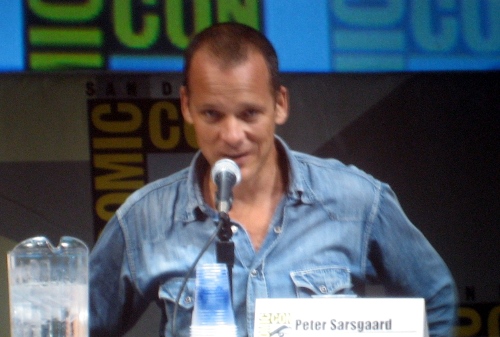In this detailed image taken at an indoor convention, likely Comic-Con, a man identified as Peter Sarsgaard sits centrally behind a microphone. He is dressed in a blue button-down shirt with the top two buttons open, speaking and looking directly ahead. In front of him, a name tag also reads "Peter Sarsgaard." The background prominently features a large poster with the words "Comic-Con" written in green and yellow letters, with "Comic" displayed vertically and "Con" horizontally across multiple rows. The top row has a blue background and green lettering, while subsequent rows mix blue with lighter yellow text, though some areas appear slightly out of focus. A pitcher of water sits on the table to Sarsgaard's right, adding to the scene's detailed setting. The color palette includes white, silver, gray, brown, light brown, yellow, green, light blue, blue, tan, and black.